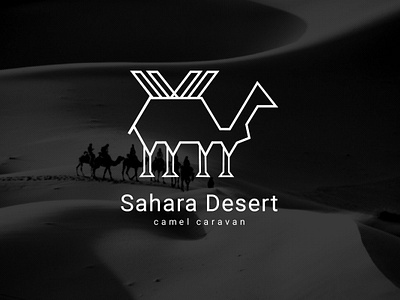The image features a dark, monochromatic advertisement for the "Sahara Desert Camel Caravan," prominently spelled out in white letters. Above the text is a simple, angular illustration of a camel in a jagged white outline with a black fill, carrying geometric cargo on its back. The backdrop showcases a serene desert landscape with swirling sand dunes, traversed by a small caravan of six camels, each carrying a rider. These camels move from left to right, casting faint trails in the sand. The overall contrast of the image is low, making the scene appear in deep shadows, with camels and dunes depicted in stark silhouette. The minimalist yet evocative composition captures the mystique and vast expanse of the Sahara Desert.